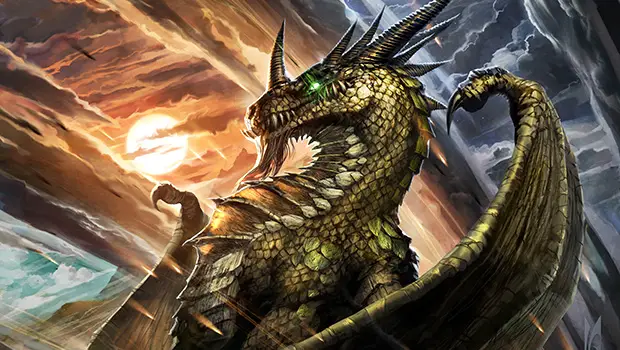This intricate illustration depicts a fearsome dragon with gold and green scales, rearing up and facing to the left. Its piercing greenish-yellow eyes glow intensely beneath a prominent horn on its nose, amidst several other horns crowning its head. The dragon brandishes immense claws, one prominently extending from its tail and another from the front of its body, while massive wings, each adorned with huge claws at the top, emphasize its formidable presence. Its maw is filled with large, sharp teeth beneath a fierce snarl, complemented by a rugged beard. The sky behind the dragon transitions from stormy blues and whites to vibrant oranges and yellows, suggesting a sun or moon partially veiled by storm clouds. Though dark and ominous above, the scene's lower half hints at serene water with shadowy mountains in the distance, all encased in an otherworldly, comic book-style aesthetic.